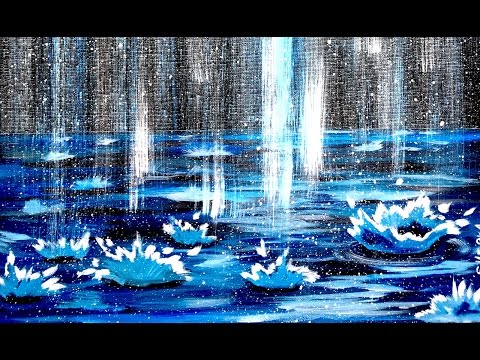This detailed description captures the essence of the painting, highlighting its key features:

"The artwork, housed in a rectangular frame about four inches wide and three inches high, features thin black bands at the top and bottom. The painting depicts a serene scene of a blue lily pond under a rainstorm. The background is a mix of blacks, whites, and blues, arranged in a cascading and interlocking vertical pattern. The main focal point consists of lighter blue lily pads with white edges, scattered across a darker blue water surface. White streaks of rain, resembling torrents, cascade down the image in columnar formations, creating splashes as they hit the water, some highlighted with white-capped tips. The interplay of colors and the fine detailing of the rain create a dynamic yet tranquil illustration of a rainy day on a lily pond."